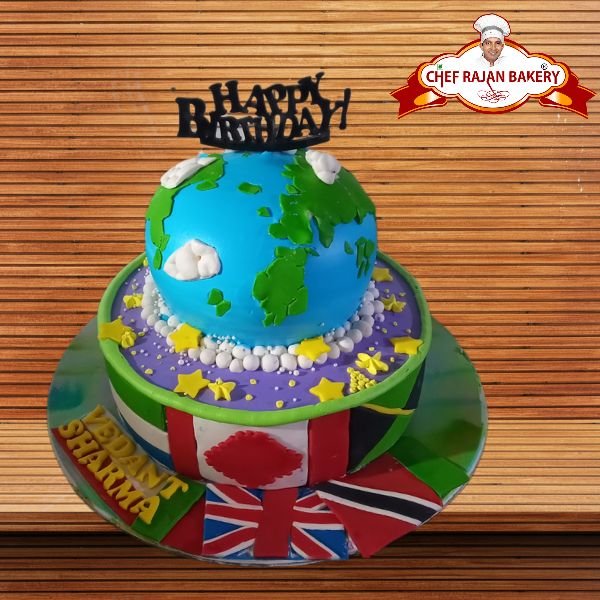In this square image, the background is made up of horizontal wooden slats in a range of brown tones. The surface on which the main object—a cake—rests appears to be composed of similar wooden slats oriented perpendicularly. 

In the upper right corner, there is a cloud-shaped logo that reads "Chef Rajan Bakery" in red text, featuring an illustration of a chef's face with a chef hat and red ribbons hanging on each side.

The centerpiece of the image is an elaborate two-tier birthday cake. The bottom tier is flat and circular, decorated with various national flags, including the British flag. A yellow bubble letter inscription reads "Vedant Sharma" on one of the sections. The second tier also features flags along its border. This tier has a purple background adorned with yellow stars and small white balls. 

Crowning the cake is a blue and green globe, with "Happy Birthday" inscribed in black at the very top. The cake is presented on a decorative circular plate, accentuating its vibrant and festive design.